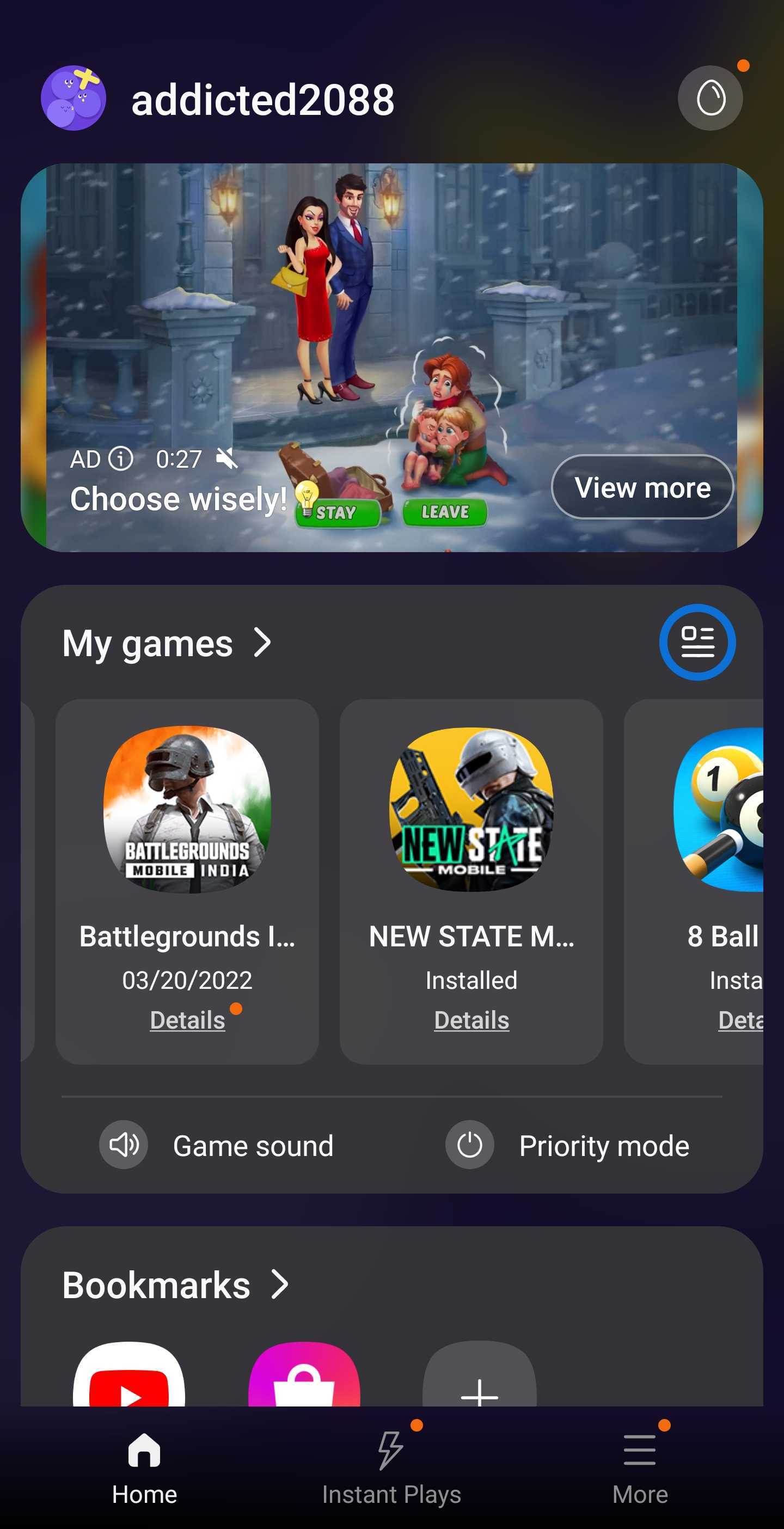Screenshot Description:

In this screenshot, a smartphone screen displays a game store or possibly a user's game library. At the top of the screen, there is a profile icon featuring three purple bowling balls arranged in a triangular pattern next to an 'X' symbol, and the username "Addicted2088". In the upper right corner, there's a water drop icon whose function is unclear.

The main focus of the screen is a promotional panel for a game depicting a dramatic scene: a man in a suit and a woman in a red dress, both looking agitated, stand in a large mansion's opulent interior. Contrasting this, another smaller image within the same panel shows a woman and two children on their hands and knees, shivering in the snow. The caption below reads, "Choose wisely: Stay or Leave," followed by an option to "View More."

Below this, the section titled "My Games" is visible, showcasing game icons. The first game listed is "Battlegrounds Mobile India," a first-person shooter. Adjacent to it is another first-person shooter, "New State Mobile." Partially visible next to these is a game with a pool theme, titled "8 Ball." 

The screen also highlights a feature labeled "Game Sound in Priority Mode," suggesting sound settings can be adjusted for a better gaming experience. At the bottom of the screen, a bookmarks tab is present, displaying icons for YouTube, a commerce site with a shopping bag on a pink background, and an option to add more bookmarks represented by a blank icon with a grey plus sign.

Lastly, at the very bottom, a navigation menu consists of various options including Home, Instant Plays, and more options to the right.